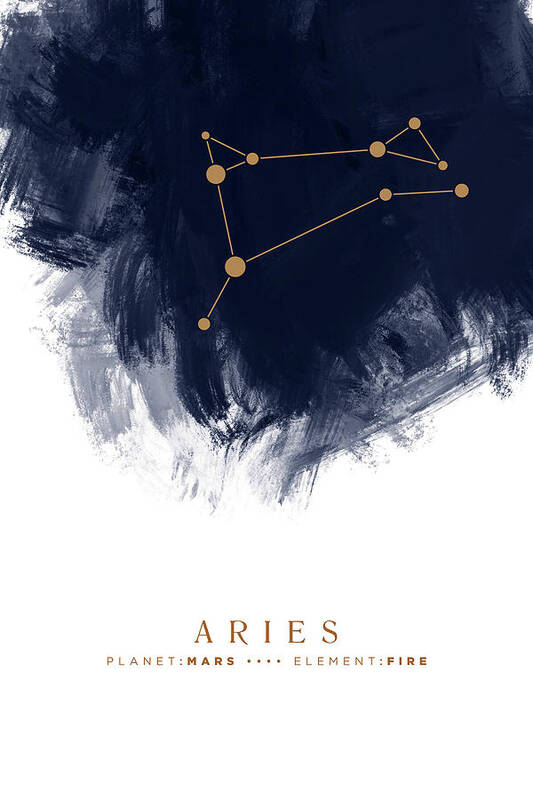This detailed and modern digital illustration of the constellation Aries features a deep blue and Payne's gray sky at the top, presented with skillful brush strokes that transition into the space surrounding the constellation. At the bottom, gold script elegantly reads "Aries, Planet: Mars, Element: Fire." The constellation itself is depicted with variously sized golden circles representing the stars that form Aries, meticulously connected by fine lines that outline the shape of the ram's horns and body. This creates a crisp and clean visual aesthetic. The background gives way to an almost cloudy texture that enhances the cosmic theme, while the use of gold against the dark, gradient background adds a striking contrast, ensuring the constellation stands out vividly. The image, in portrait format, successfully combines a modern artistic approach with the timeless allure of celestial navigation.